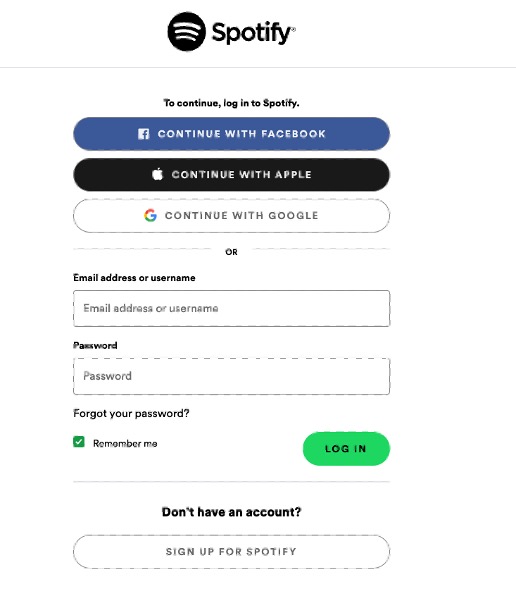This is a detailed screenshot of the Spotify login page on a desktop browser. At the top center of the page, the well-known Spotify logo is prominently displayed. Just below the logo, the header prompts users to continue by logging in to Spotify. 

Three prominent buttons are aligned vertically below the header, offering users different login options. The first option, "Connect with Facebook," is highlighted in blue. Directly beneath it, a black button offers the "Connect with Apple" option, followed by a white button for "Connect with Google." 

An alternative login method is suggested with the text “or, you can add in your email address or username and password." Below this text, there are two input fields for the user's credentials. Adjacent to these fields, a link is provided for users who have forgotten their password.

A "Remember me" checkbox, marked with a green checkmark, indicates that the feature is enabled. Positioned to the right of these options, a green "Log In" button invites users to proceed. 

At the bottom of the screen, it addresses new users with the text, “Don’t have an account? Sign up for Spotify.” A large, white button is available for new users to create an account. 

The overall page design is clean and functional, featuring a predominantly white background with all text rendered in a black font, clearly indicating this is likely a desktop version of the Spotify site.